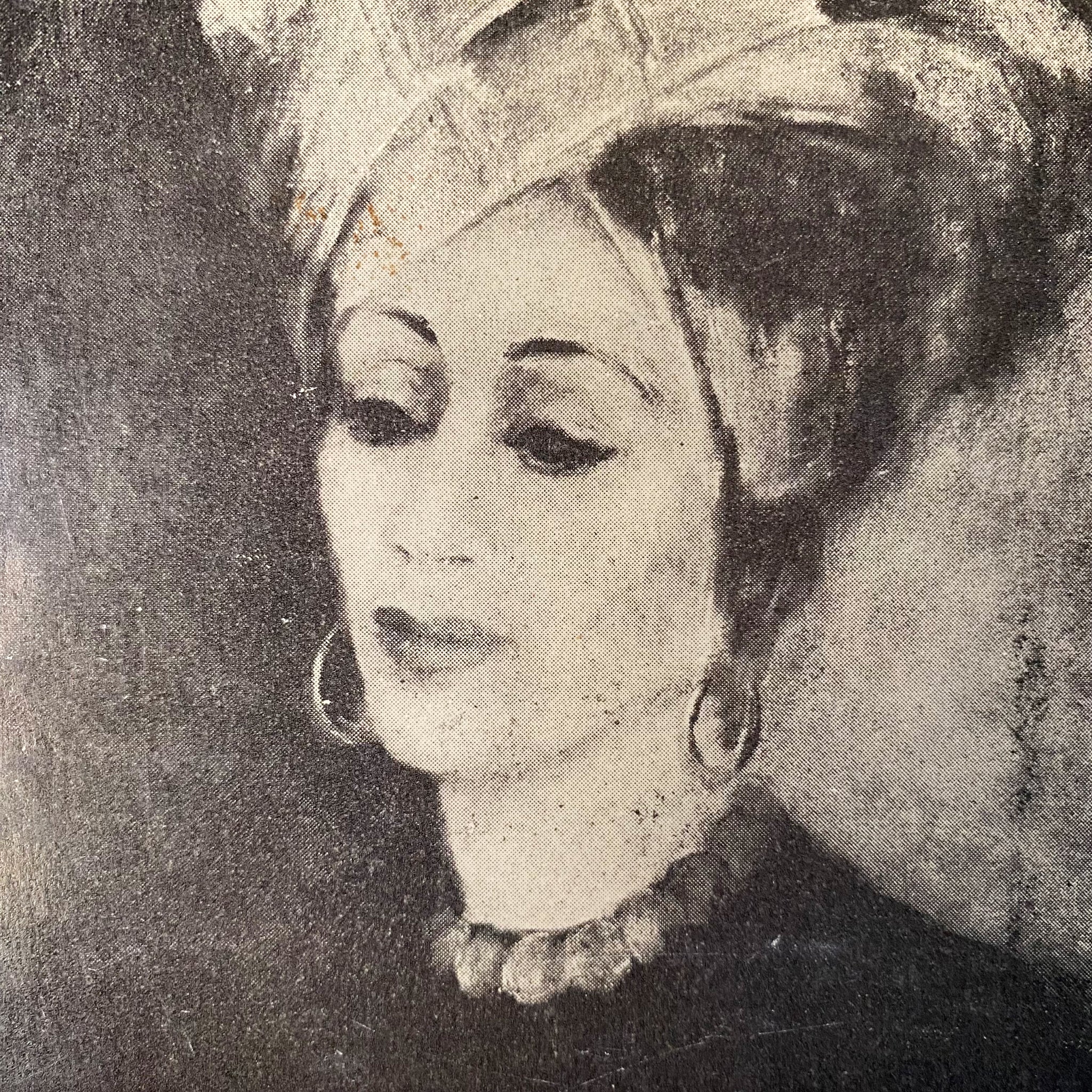This black and white image, resembling a photocopied or printed version of a painting or charcoal drawing, portrays a woman of fair complexion. Her face, elaborately made up with eye shadow, lipstick, and thin, arched eyebrows, suggests a well-groomed appearance. She dons a thick, pearl-like bead necklace tightly around her neck and large, hoop earrings. Her hair is styled up, wrapped in a voluminous fabric turban or headdress, adding to her elegant aura. The image, which is a vertically oriented rectangle, crops her just below the shoulders, placing her at the center. She is facing left with her gaze lowered. The background appears grainy and fuzzy, with a predominantly gray tone; it is darker on the left side, transitioning to a lighter shade on the right.